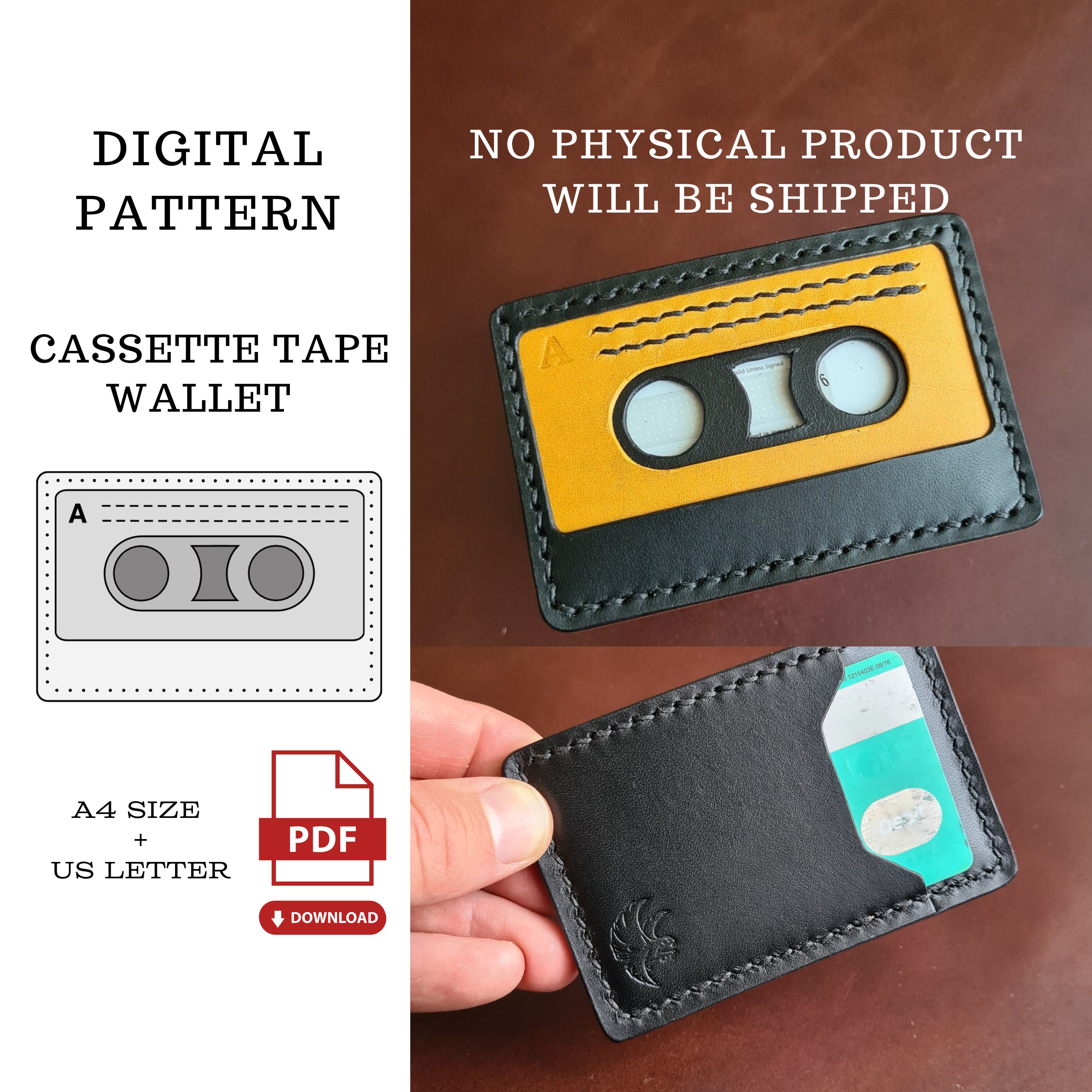The advertisement showcases a digital pattern PDF for creating a cassette tape wallet. The image is divided into two main sections. On the left, there is a white background with black text. It prominently displays "Digital Pattern Cassette Tape Wallet," accompanied by a picture of a wallet resembling a cassette tape, annotated with details like "Side A" and specifications for "A4 Size plus U.S. Letter patterns."

On the right side, occupying the majority of the image, there is a brown, desktop-like background featuring two images of the wallet. The upper segment states, "No Physical Product Will Be Shipped" in bold white letters. It displays the front of the wallet crafted in black and yellow leather, detailed with sewing lines, two circular holes, and a labeled "Side A." The lower segment showcases the back of the wallet, which includes a pocket holding a blue-green credit card with a white stripe. This visual representation emphasizes the intricate design and practical use of the wallet, ideal for enthusiasts of retro cassette tape aesthetics.